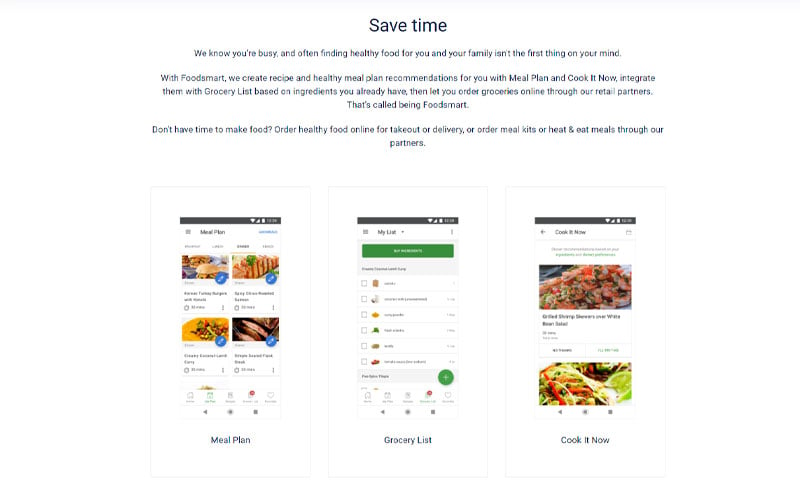This image showcases screenshots from a meal planning app set against a solid white background. The prominent black text at the top reads: "Save time. We know you're busy and often find healthy food for you and your family isn't the first thing on your mind. With Food Smart, we create recipe and healthy meal plan recommendations for you with meal plan and cook it now, integrate them with a grocery list based on ingredients you already have, and then let you order groceries online through our retail partners. That's called being Food Smart. Don't have time to make food? Order healthy food online for takeout delivery or order meal kits or heat-and-eat meals through our partners."

Below this comprehensive statement, there are three distinct phone screenshots aligning horizontally. 

1. The screenshot on the left, titled "Meal Plan," displays four different meal plan options, each with accompanying imagery.
2. The middle screenshot, titled "Grocery List," shows a detailed grocery list interface, complete with checkboxes next to each item. A green button and the text "My List" are visible above the checklist.
3. The screenshot on the right, titled "Cook It Now," features images of a shrimp dish and a taco or fajita dish, reflecting options for immediate cooking.

Each screenshot includes the typical phone navigation bar at the top, displaying cell signal strength, Wi-Fi status, the current time, and battery life. This cohesive structure provides a clear, detailed view of the app’s functionalities and ease of use, making meal planning and grocery shopping more efficient for busy individuals.